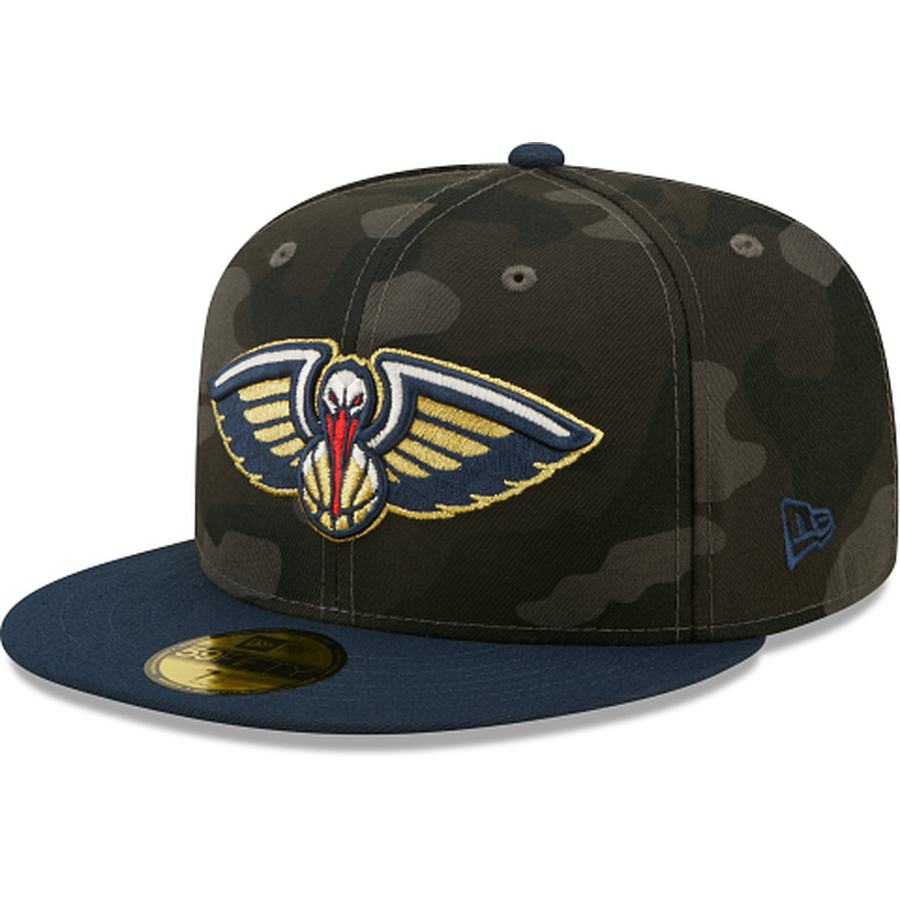The image showcases a new New Orleans Pelicans basketball cap set against a stark white background. The cap is positioned diagonally to the left, emphasizing its clean, modern design. The brim is a dark navy blue, and a gold and black sticker is affixed in the center, highlighting its pristine condition. The hat's crown features a dark green and gray camouflage pattern. Centrally, the New Orleans Pelicans emblem stands out prominently: a white pelican head with a striking red beak topping a basketball. The pelican's large wings curve gracefully upward around the head, adorned with gold horizontal streaks and blue outlines, accentuated by yellow and white borders. On the bottom right of the cap, the manufacturer's logo is displayed on a small blue flag. A subtle shadow beneath the cap suggests professional editing, enhancing the crisp presentation of the hat.